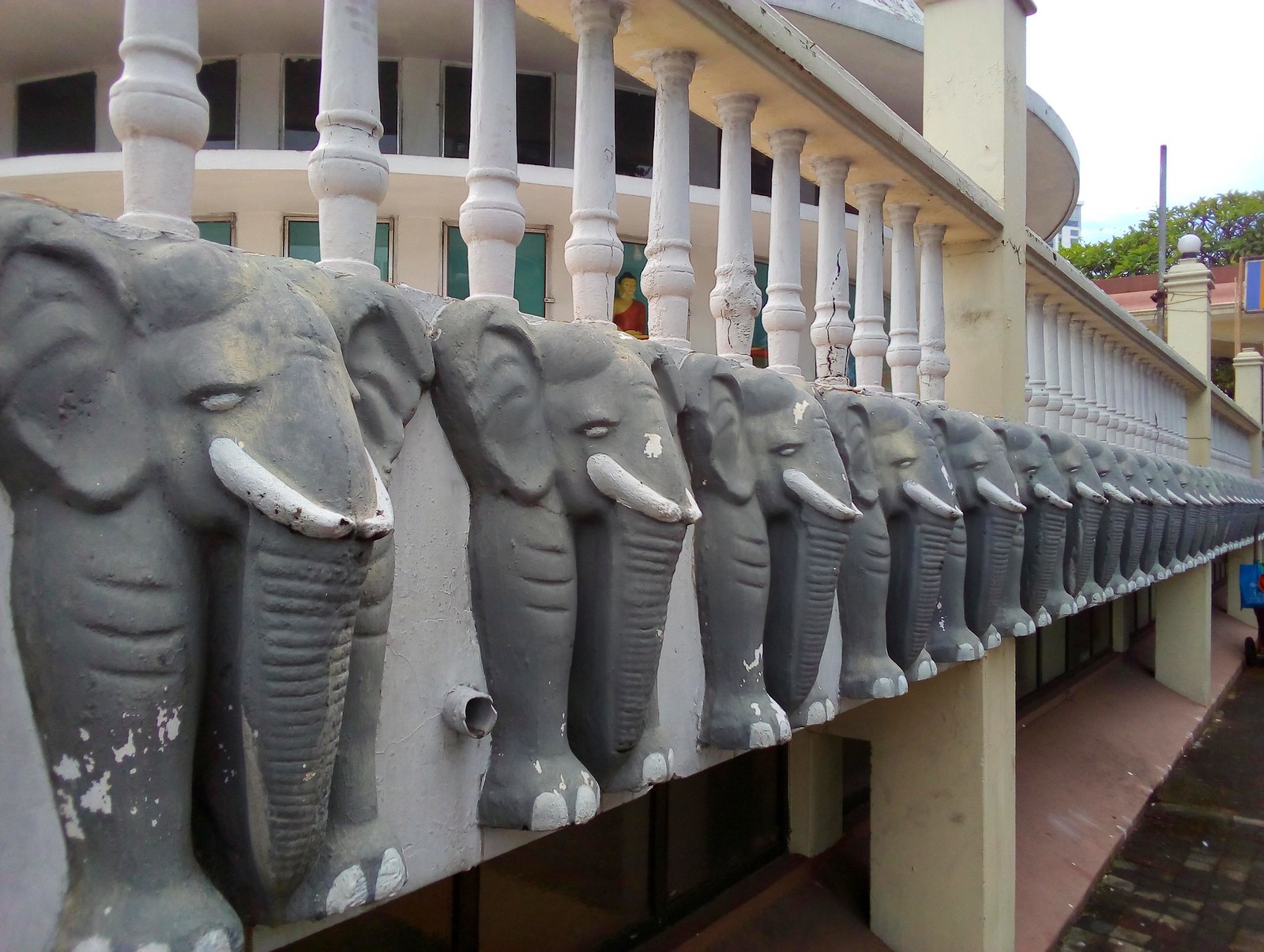This outdoor photograph captures a detailed scene of a distinctive balcony adorned with elephant sculptures. Dominating the immediate foreground is a white-railed balcony featuring approximately 20 to 30 gray elephant sculptures with white tusks. These sculptures, depicting only the elephants' heads, ears, trunks, and front legs, are intricately carved yet show signs of wear and chipping paint. The spindles and posts of the railing are also white, complemented by a light yellow handrail that runs along the top.

The background reveals a cluster of green trees and a partly white sky in the top right corner, suggesting a bright, yet somewhat overcast day. At the center of the background stands a prominent circular building with a white frame and windows encircling its structure, contributing an exotic architectural element that may hint at influences from countries like Thailand. The elephants seem to be integrated into a second-floor structure, giving the balcony a unique and internationally inspired aesthetic. The entirety of the scene is urban, suggesting it is part of a well-aged, potentially historical, city setting.